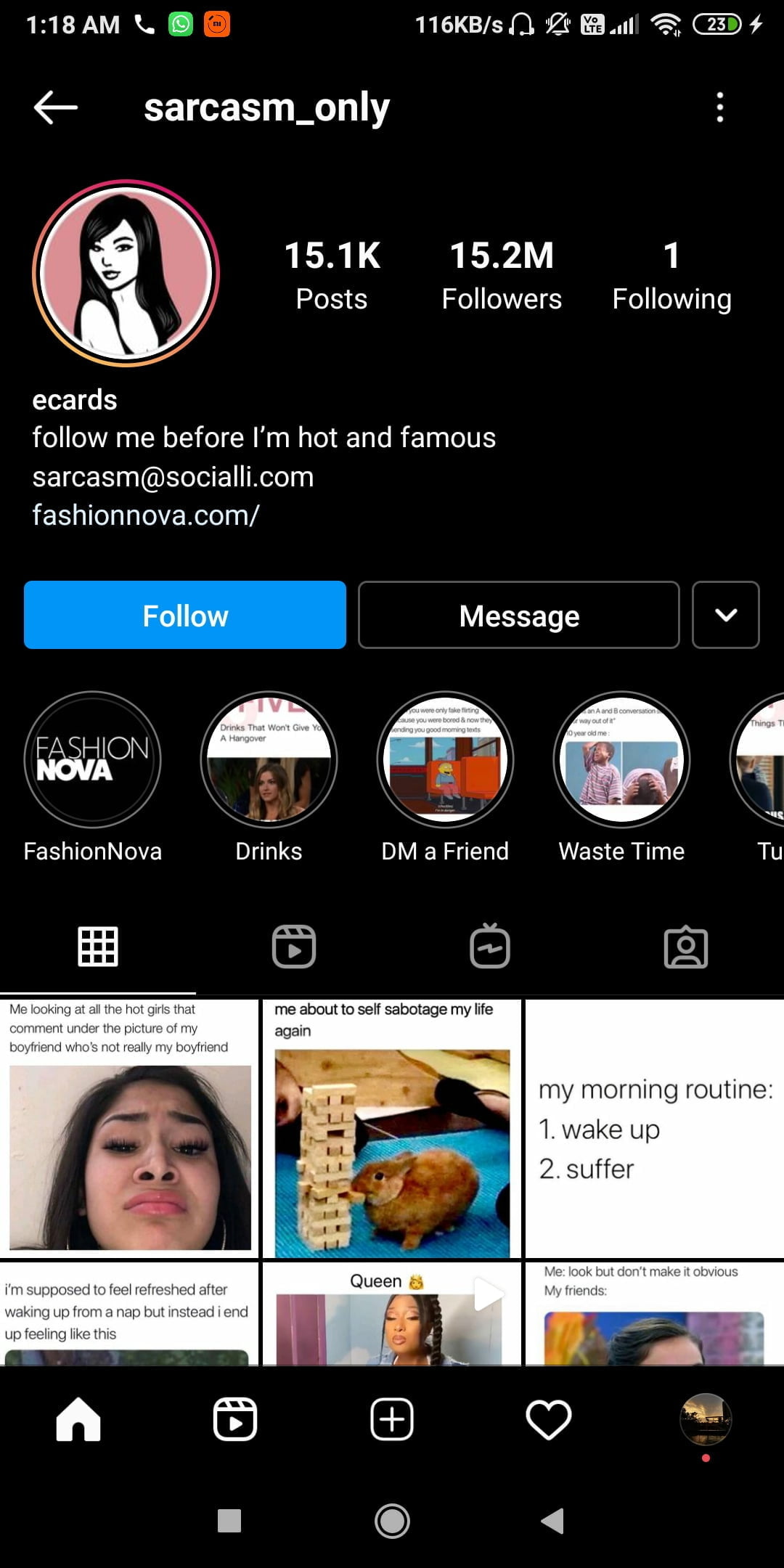The image is a mobile device screenshot taken at 1:18 a.m. featuring a black background. At the top of the screen, the status bar displays various icons: the WhatsApp logo in green next to an alarm bell, near-full carrier signal strength, enabled Wi-Fi, and a battery at 23% currently charging. Additionally, a white arrow indicator is present.

Below the status bar, the screenshot reveals what appears to be an Instagram profile named "sarcasm_only." The profile picture is circular with a pink background portraying a cartoon-like image of a woman with dark hair and a white face and body. The account statistics show 15.1 thousand posts, 15.2 million followers, and follows only one other account.

The profile description humorously reads, "Follow me before I'm hot and famous," and it references an e-card with the caption "Sarcasm at socialally.com". Additionally, there's a mention of the website "fashionnova.com."

The profile also displays several story bubbles with titles like "Waste Time," "DM a Friend," and "Drinks," indicating different categories of posts the user has shared.